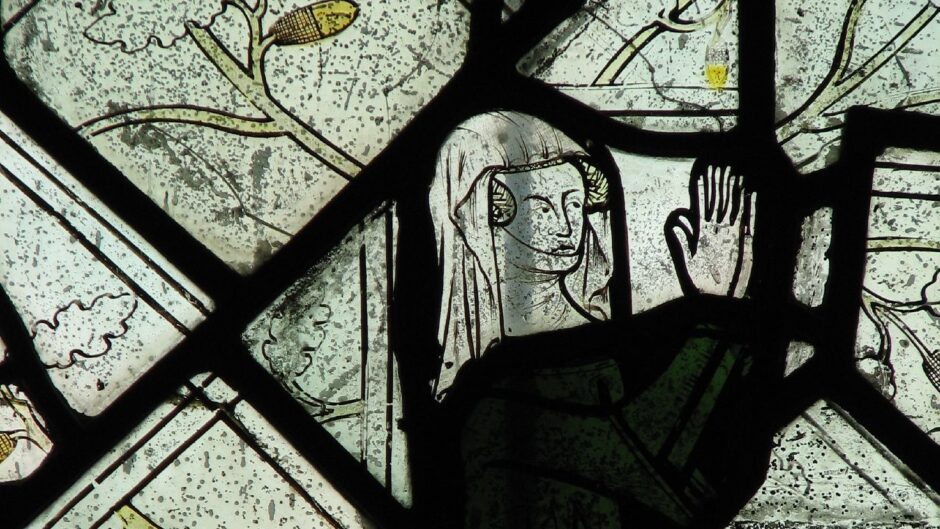The artwork resembles a stained glass window, depicting a woman in deep prayer, her hands clasped together. She wears a white veil over her head, similar to that of a nun, with rounded braids visible near her temples. A dark green robe covers her body, adding a muted splash of color to the primarily black and white composition. Her face, rendered minimalistically, shows a serious expression, capturing the essence of solemn prayer. The artwork is divided into sections by black lines, reminiscent of a stained glass window, with each section containing different scenes like tree trunks, limbs, and elements of nature. There are subtle hints of yellow in certain quadrants, with one corner featuring a branch with an acorn. The divisions have no specific pattern, contributing to the abstract, almost modern art or Picasso-like feel of the piece. Overall, the detailed portrayal of the praying woman, the intricate natural elements, and the abstract division of the background create a thoughtfully crafted and evocative image.